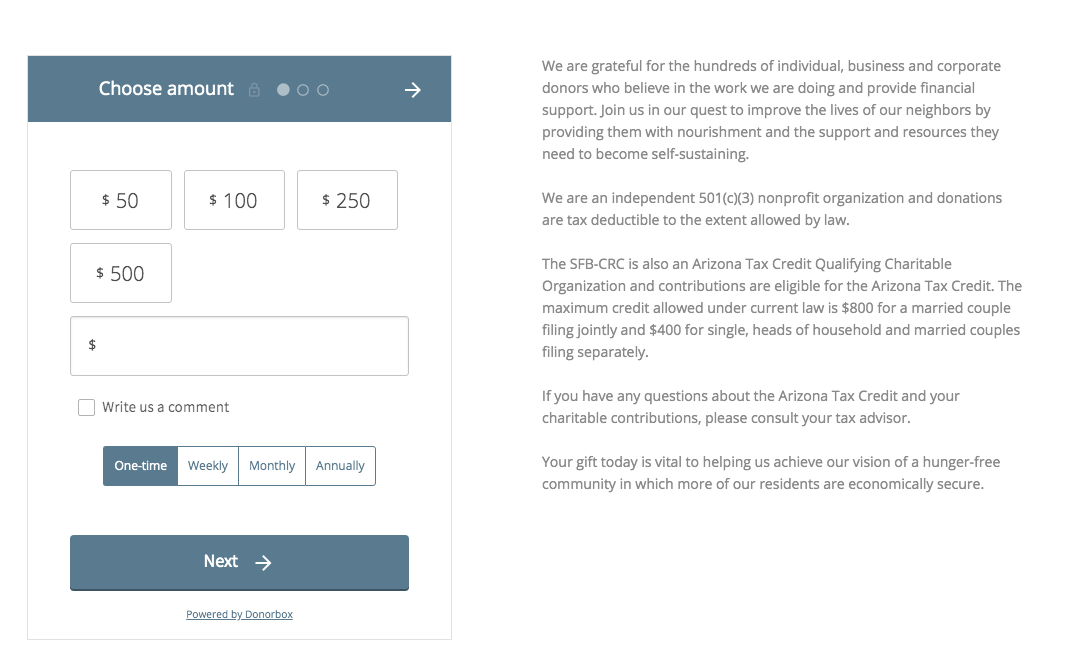The image is divided into two sections. On the left-hand side, there is a detailed graphic of a donation interface, while the right-hand side contains a disclaimer for a tax-qualifying donation. The entire graphic is enclosed within a light gray border.

The interface begins with a blue-gray banner at the top that reads "Choose Amount" in white text, accompanied by a small, very light gray lock icon. Beneath the banner are three gray elements; a dot followed by two gray-outlined circles, and a white arrow pointing to the right. 

Below this section, there are three equally sized gray-outlined rectangles displaying preset donation amounts: $50, $100, and $250. Following this row is a single gray-outlined rectangle labeled $500. Further down, there is a longer gray-outlined rectangle with a dollar sign inside, which is left blank for custom entry.

Continuing downward, there is a small gray-outlined square box that prompts "Write us a comment." 

Below the comment box, there are four option buttons: "One Time," which is grayed out, "Weekly," "Monthly," and "Annually." 

At the bottom of the interface is a large gray button that says "Next," paired with a forward-pointing arrow, and the phrase "Powered by DonorBox" at the bottom of the screen.